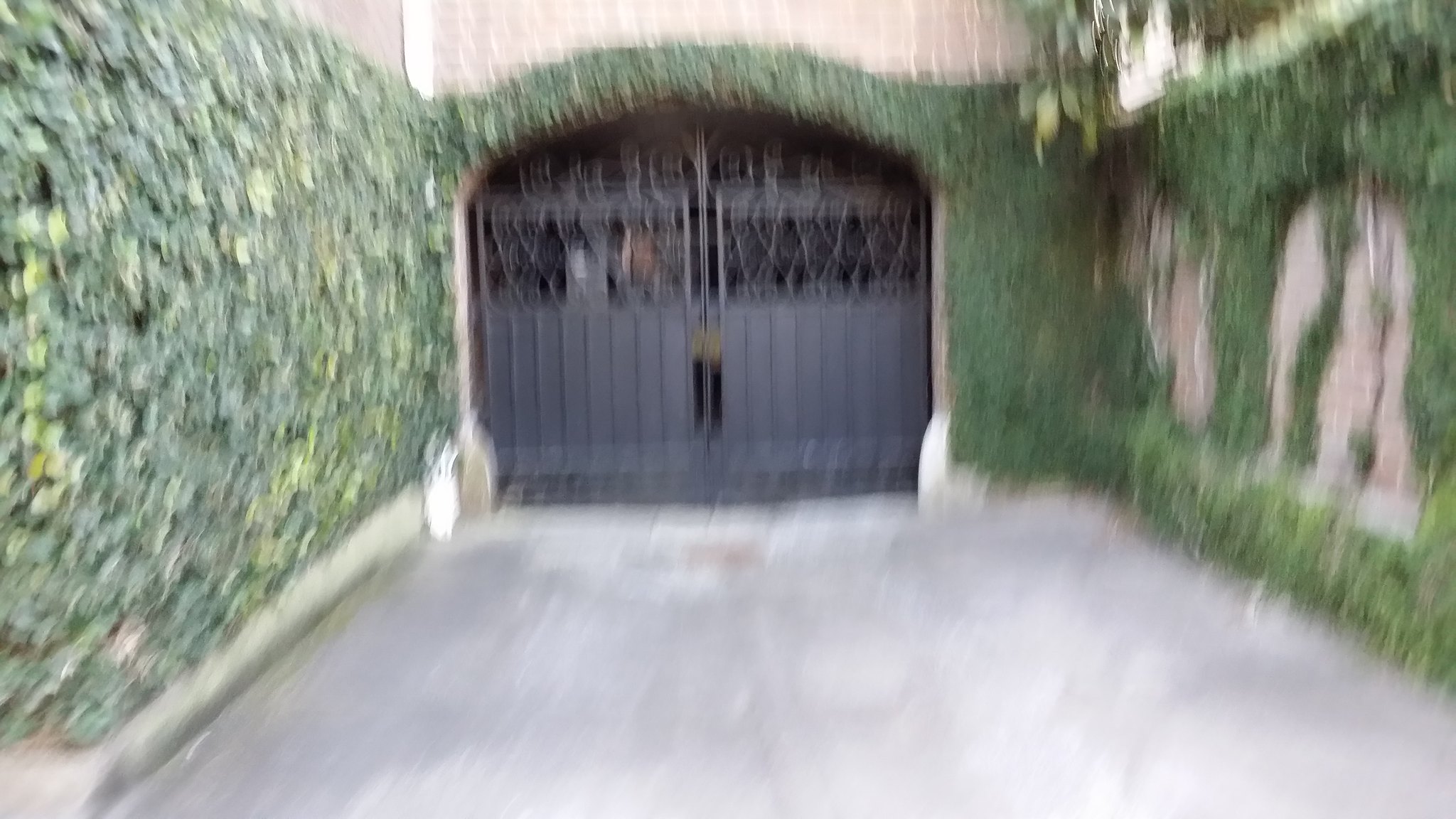This blurry image captures the entrance to a garage, framed by an iron gate with an intricate design on its upper half. The iron gates, meeting in the middle under an archway, are shrouded in a lush blanket of green ivy that extends over the surrounding walls. The camera movement when the photo was taken adds a sense of urgency or motion, further softening the view of the driveway and the road leading up to the entrance.